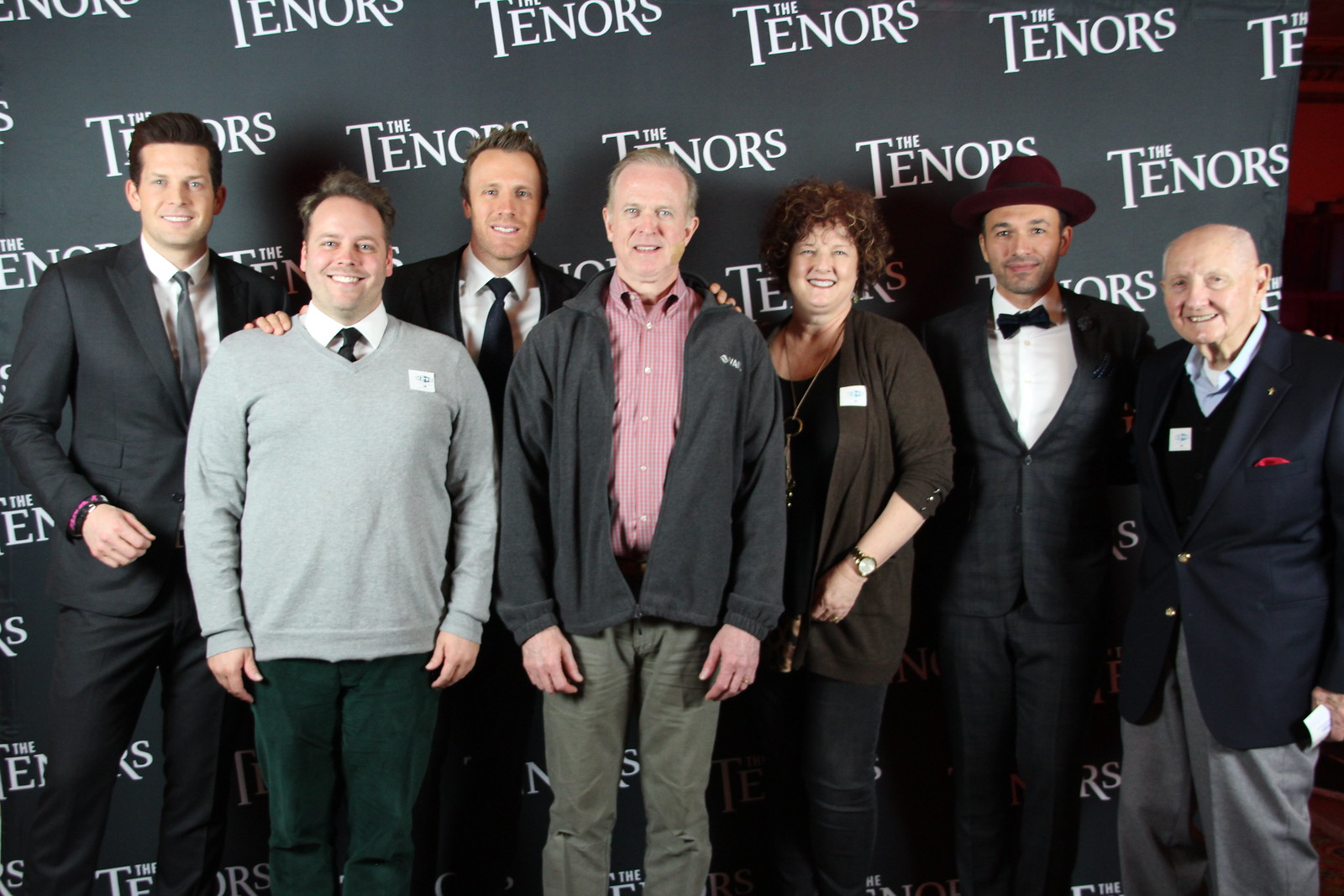Seven individuals, comprising six men and one woman, stand in front of a black banner featuring the word "The Tenors" repeatedly in white text. From left to right, their attire varies but maintains a formal tone. The first man, with short brown hair and fair skin, wears a dark suit with a white shirt, grey tie, and a pink wristband. He rests his hand on the shoulder of the second man, who has short, slightly balding brown hair and also fair skin. This man is dressed in a grey sweater over a white collared shirt and black tie, accompanied by green pants.

Behind him is a man with longer, lighter hair, dressed in a black suit jacket, white shirt, and black tie. He places his hand on the shoulder of the fourth person, an older man with a somewhat awkward smile, wearing a black zip-up fleece jacket over a red and white striped buttoned shirt and light green pants. 

Next to this older man stands a woman with very curly brown hair. She is dressed in a brown sweater over a black top, adorned with either jewelry or a lanyard around her neck, black pants, and a wristwatch.

To her right, a man in a tuxedo with a faint plaid pattern stands out, accentuated by a black bow tie and a small red-brimmed hat. Lastly, the final person in the lineup is a very elderly man with hunched shoulders, dressed in a suit jacket with a red cloth in the breast pocket, a black sweater, a blue button-up shirt, grey pants, and holding something in his hand. Some individuals have their hands on others' shoulders, adding a sense of camaraderie to the group photograph.